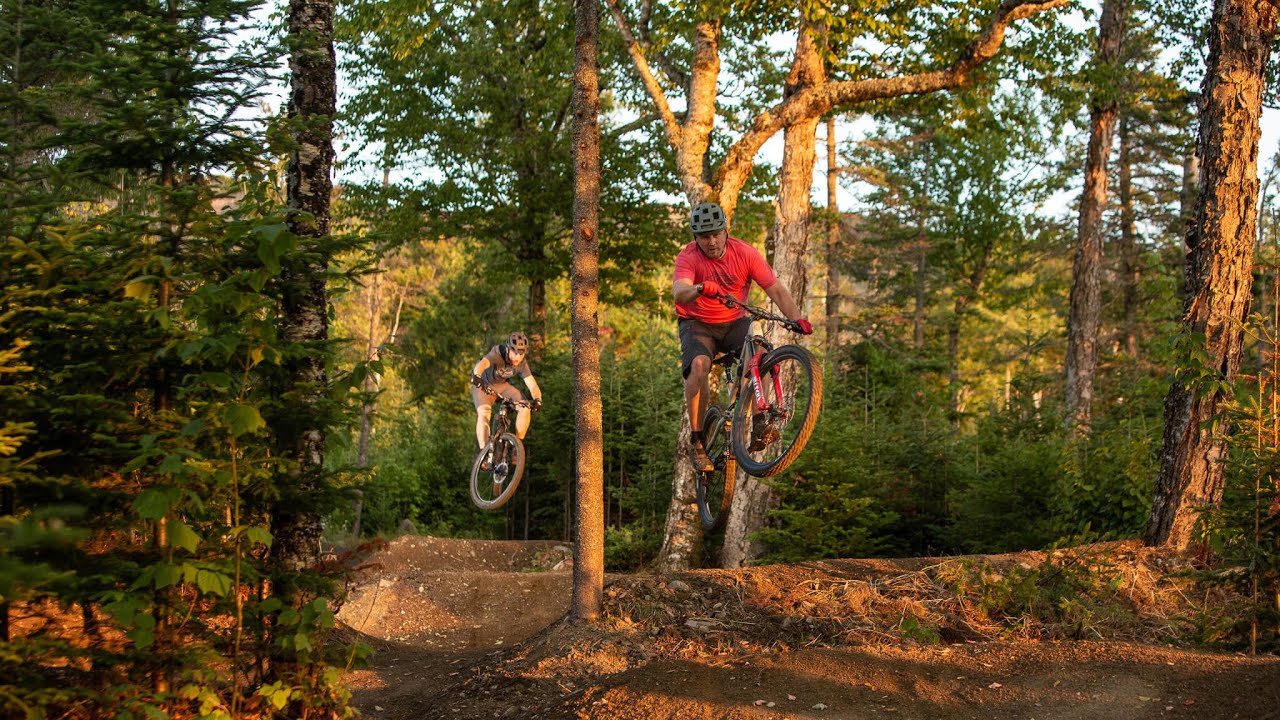In this dynamic and detailed outdoor image, two mountain bikers are captured mid-air after launching off dirt ramps on a well-worn forest trail. The foreground focuses on six tree trunks, with a mix of adult trees towering off-screen and a smaller, younger tree about six to eight feet tall. Yellow, green leaves and scattered branches add to the dense foliage, which trails off into a mix of deciduous and pine trees highlighted against a blue sky filled with a few clouds.

The leading biker, front and center, is easily identifiable by his red shirt, black shorts, and grey helmet. His bike, predominantly red, matches his red gloves and black pants. He appears about a foot off the ground with his front tire lifted and handlebars slightly cocked to the left. 

Immediately behind him, another biker, dressed in a black shirt and black shorts with visible white socks, mirrors his airborne stance on a black bike. Both riders are clearly experienced, their helmets and gear appropriate for the rugged, off-road terrain.

The photo captures the thrill of their ride through a serene, picturesque forest with detailed, papery bark on the trees and a dirt trail strewn with roots and leaves. This snapshot in time beautifully conveys the excitement of mountain biking amidst nature's verdant embrace.